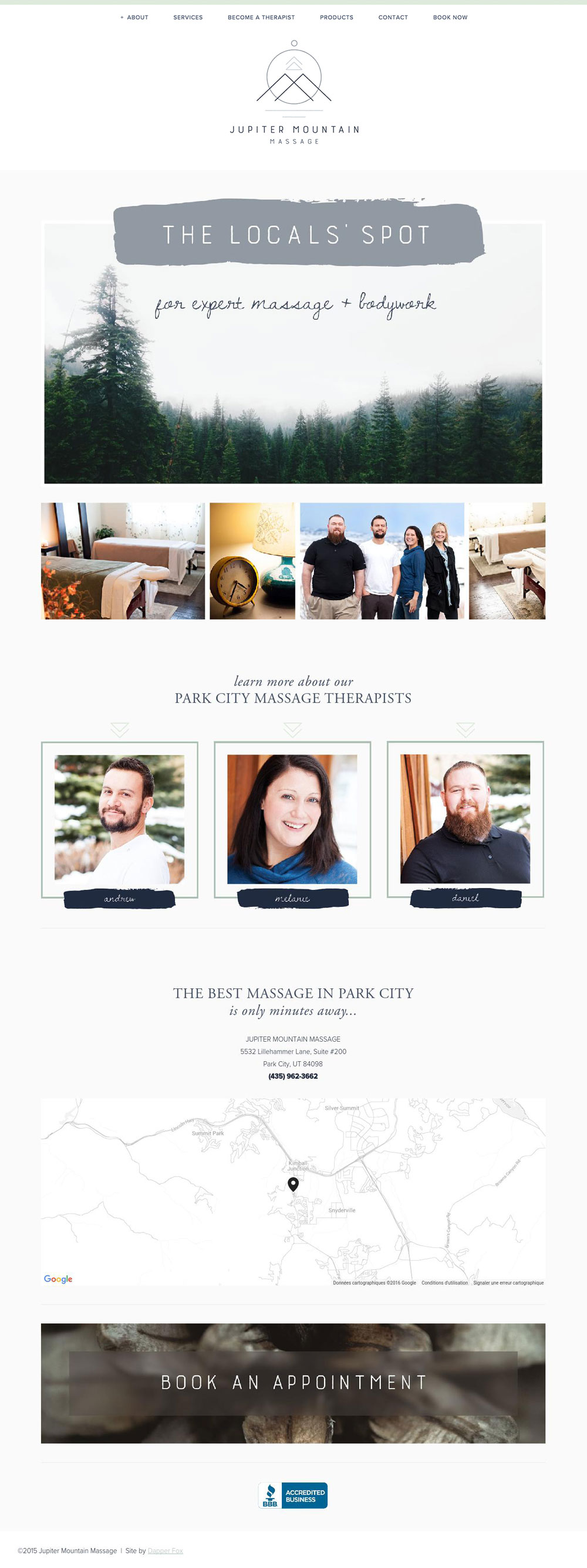**Screenshot of Jupiter Mountain Massage Business in Park City, Utah**

The screenshot features promotional content for Jupiter Mountain Massage, a massage and bodywork business located in Park City, Utah.

At the top center of the vertically oriented screenshot, there is a logo composed of two interlocking upside-down "V" shapes, representing mountains, with a circle traversing the top of the mountain shapes. Below this emblem, the name "Jupiter Mountain Massage" is prominently displayed.

In the upper center of the screenshot, a rectangular photograph showcases a picturesque mountainous landscape with lush green pine trees in the foreground. At the top of this photograph, within a gray oval-shaped overlay, the text "The Locals Spot" is inscribed with the phrase "For Expert Massage and Bodywork" positioned just below it.

Beneath the main photograph, there is a horizontal array of four smaller images: 
1. A beautifully arranged massage room.
2. A close-up of a clock and a lamp.
3. A group of four individuals, comprising two males and two females.
4. The lower half of massage beds.

Centered below these images is the inviting text: "Learn More About Park City Massage Therapists."

Further down, three square photographs depict the massage therapists at Jupiter Mountain Massage:
1. On the left, a male therapist with short, dark hair, a mustache, and a beard, wearing a white shirt. He is looking directly at the viewer while his body faces slightly to the left.
2. In the center, a female therapist with shoulder-length dark hair and light skin, smiling warmly with her head tilted slightly to the right.
3. On the right, a male therapist with red hair, short beard, and mustache. He is tilting his head slightly to the left, looking straight ahead.

This well-arranged screenshot effectively highlights the professionalism and inviting nature of Jupiter Mountain Massage, setting an appealing tone for potential clients.